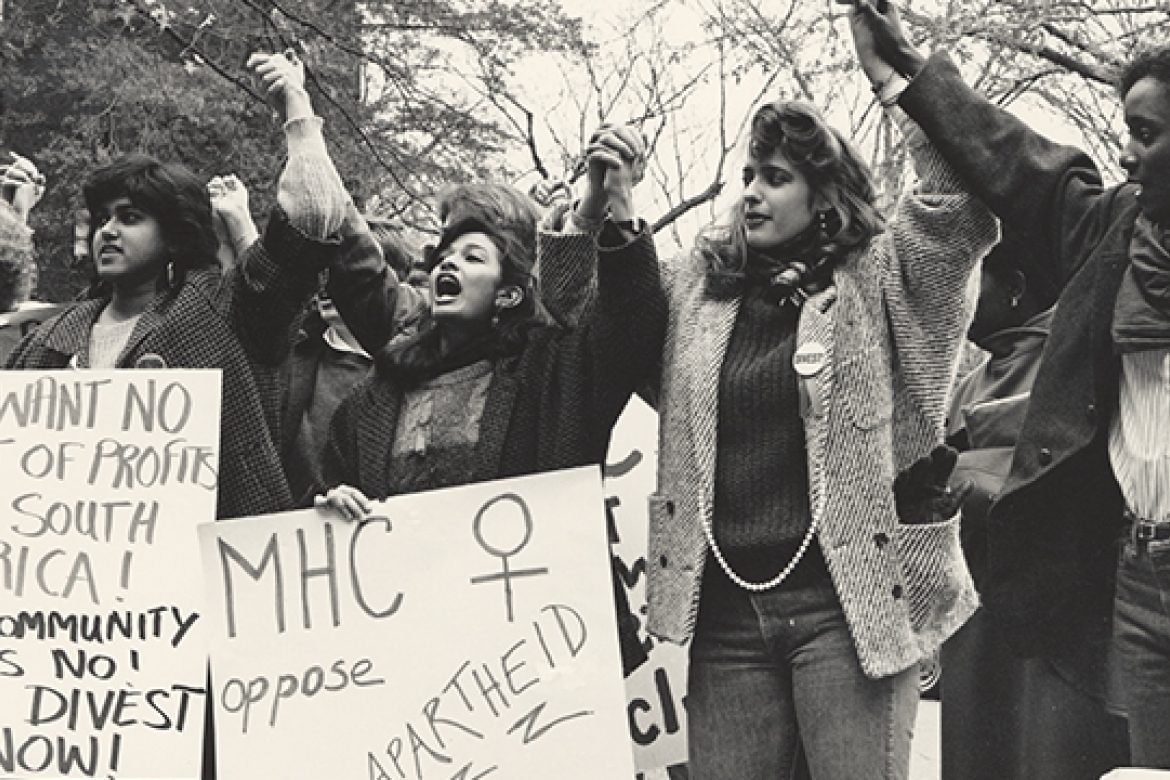This black-and-white photograph captures a powerful protest scene featuring a diverse group of women standing in unity. The focal point is a row of women, each raising their hands interlocked in solidarity, while behind them, more protesters mimic the same gesture. Ethnic diversity is evident, with visible Hispanic, African American, and Caucasian women among the front row. Two prominent signs on the left side of the image demand attention: the far-left sign, written in large letters with a magic marker, partially reads "know something of profits... South Africa... community, know... divest now." The adjacent sign to its right, featuring the letters "MHC" and the female gender symbol, clearly states "Oppose Apartheid." The attire suggests cold weather; the women are dressed in heavy jackets. Amidst the chanting and unity, trees and the sky form the backdrop, highlighting the outdoor setting of this historic protest, possibly advocating against South African mining practices.